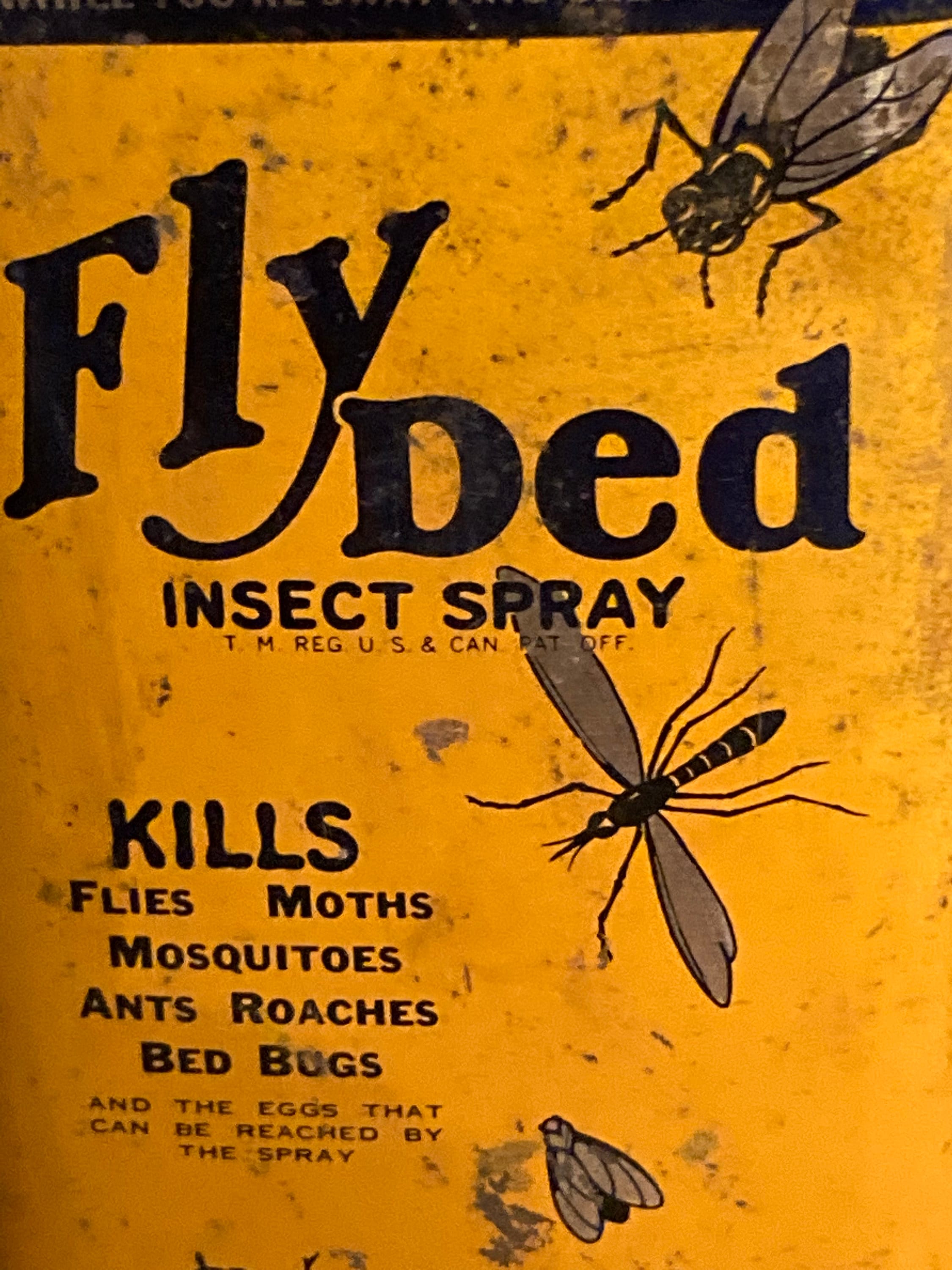This is a close-up photograph of an insect spray label, which appears to be vintage and slightly worn. The label features a bright yellow background with black font and illustrations. Dominating the top of the label are the bold, black words "FLY DED" in large letters, with "DED" spelled D-E-D. Below this, in smaller block capitals, it states "INSECT SPRAY." Further down, it includes the note "Trademark Registered U.S. and Canadian Patent Office." Surrounding this text are illustrations of various flying insects: a gray housefly at the top right, an insect resembling a mosquito with a black body off to the middle right, and a gray moth with a black rear at the bottom center. In the lower left corner, the label pronounces in fairly large uppercase font "KILLS" followed by a list in smaller font that reads: "flies, moths, mosquitoes, ants, roaches, bed bugs," and in much smaller print, "and the eggs that can be reached by the spray." The label also has a subtle black border at the top.